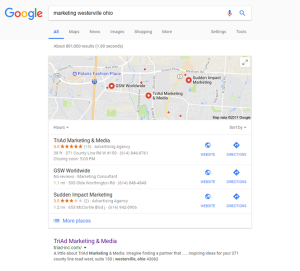A detailed screenshot of a Google search results page. The iconic Google logo is prominently displayed in the top left corner, adjacent to a search bar. While the specific keywords typed into the search bar are somewhat blurry, the last discernible word appears to be "Ohio." Below the search bar are several category tabs, including "All," "Maps," and others that are too indistinct to read. The "All" tab is highlighted in blue, indicating it is the selected category.

The main content of the page features a map showing three marked locations. Beneath the map, detailed information about these locations is provided, albeit with some parts indistinct. The first business listing has a five-star rating based on 11 reviews, accompanied by an address and operating hours. On the far right of this listing, website and directions icons are visible.

The second business, although its name is blurred, seems to be "GSW Worldwide." This listing follows a similar layout, with website and directions icons to the right.

The third row features "Sudden Impact Marketing," which holds an approximate three-star rating. Again, website and directions icons are present to the right of this entry.

Outside of this main content box, a separate link is visible labeled as "Triad Marketing and Media."